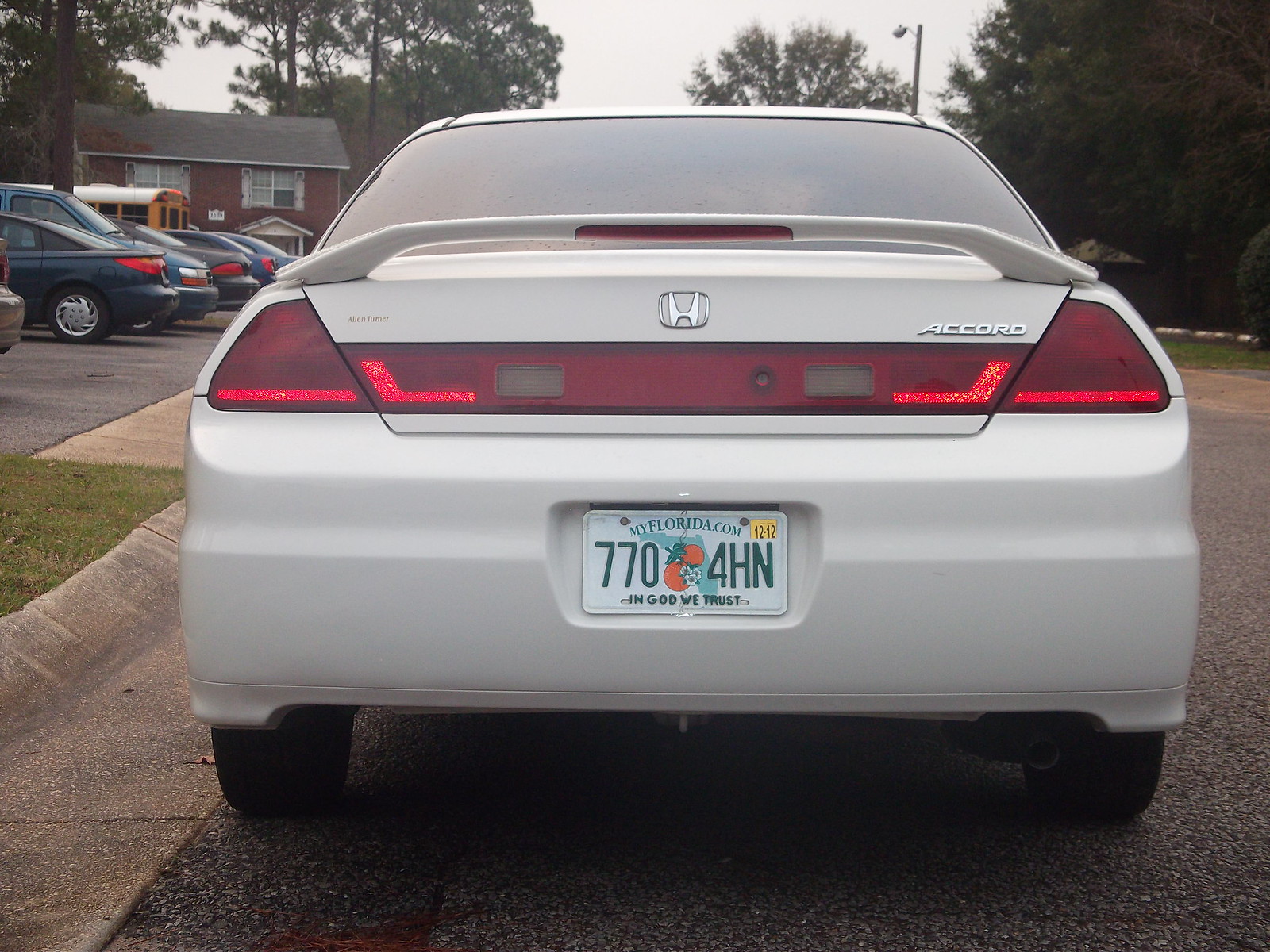This detailed horizontal photograph showcases the back of a white Honda Accord car parked on a street, prominently featuring its Florida license plate, "7704HN," adorned with the state image, two oranges, and white flowers. The tag also displays "MyFlorida.com" at the top and "In God We Trust" at the bottom, with a yellow tag positioned in the top right corner. The vehicle's silver "Accord" branding and Honda emblem are clearly visible above its red taillights, which frame the rear trunk area. The scene includes a row of parked cars to the left, including a blue car, a blue van, and a black car, leading up to a yellow school bus. Behind the row of vehicles, a reddish brick building, likely an apartment or home, is visible, along with tall green trees and patches of grass, suggesting an outdoor, urban setting.